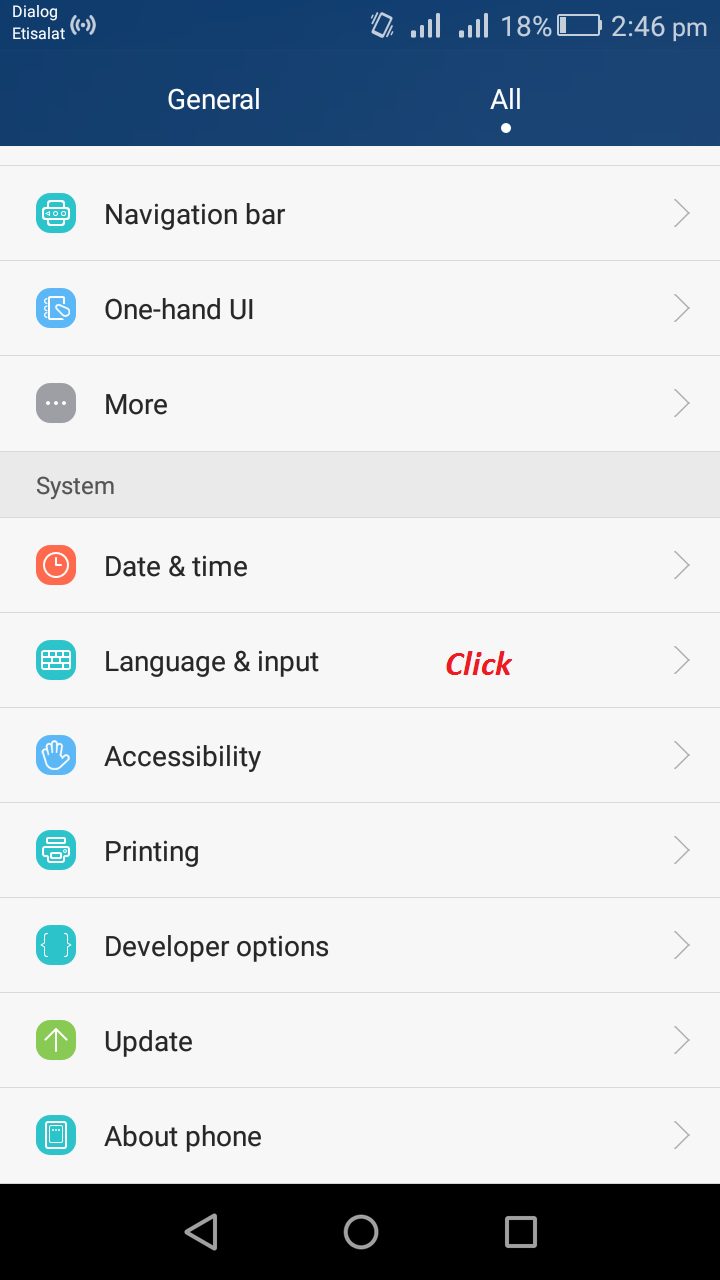This is a detailed screenshot of a settings page interface. The top of the screenshot features a prominent blue bar, with the word "General" on the left side and "All" on the right side in white text. The "All" option is highlighted by a small white dot underneath. Below this bar, the settings are divided into two main sections, each listed item accompanied by colorful icons on the left and the corresponding text on the right.

In the first section, the following options are listed: 
1. "Navigation Bar" 
2. "One-Hand UI" 
3. "More"

The second section, titled "System," includes additional settings, each set against a gray bar backdrop. The listed options are:
1. "Date and Time"
2. "Language and Input" (highlighted in red)
3. "Accessibility"
4. "Printing"
5. "Developer Options"
6. "Update"
7. "About Phone"

Each entry within these sections has a forward arrow icon on the right side to indicate further navigation options and is separated by thin gray lines for clarity.